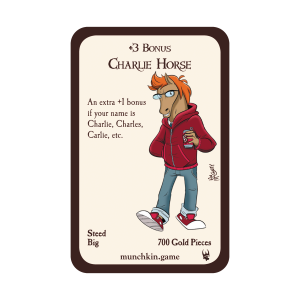This image appears to be a detailed playing card from the game "Munchkin Dot Game," featuring a cartoon character with a horse's head and a human body. The card has a dark brown border with a light tan background. Dominating the right side, the character, named Charlie Horse, is a horse-headed figure with an orange mane wearing black-framed glasses. His attire includes a red zip-up hoodie with two pockets, blue jeans, and red and white sneakers. He is depicted holding a can, possibly soda or beer, in his left hand. 

The top section of the card reads "3 BONUS CHARLIE HORSE," while the left side notes, "An extra plus one bonus if your name is Charlie, Charles, Carly, etc." At the bottom left corner, it says "STEED BIG," and the bottom right corner indicates "700 GOLD PIECES." The central part of the card is marked with the game's branding, "MUNCHKIN DOT GAME."